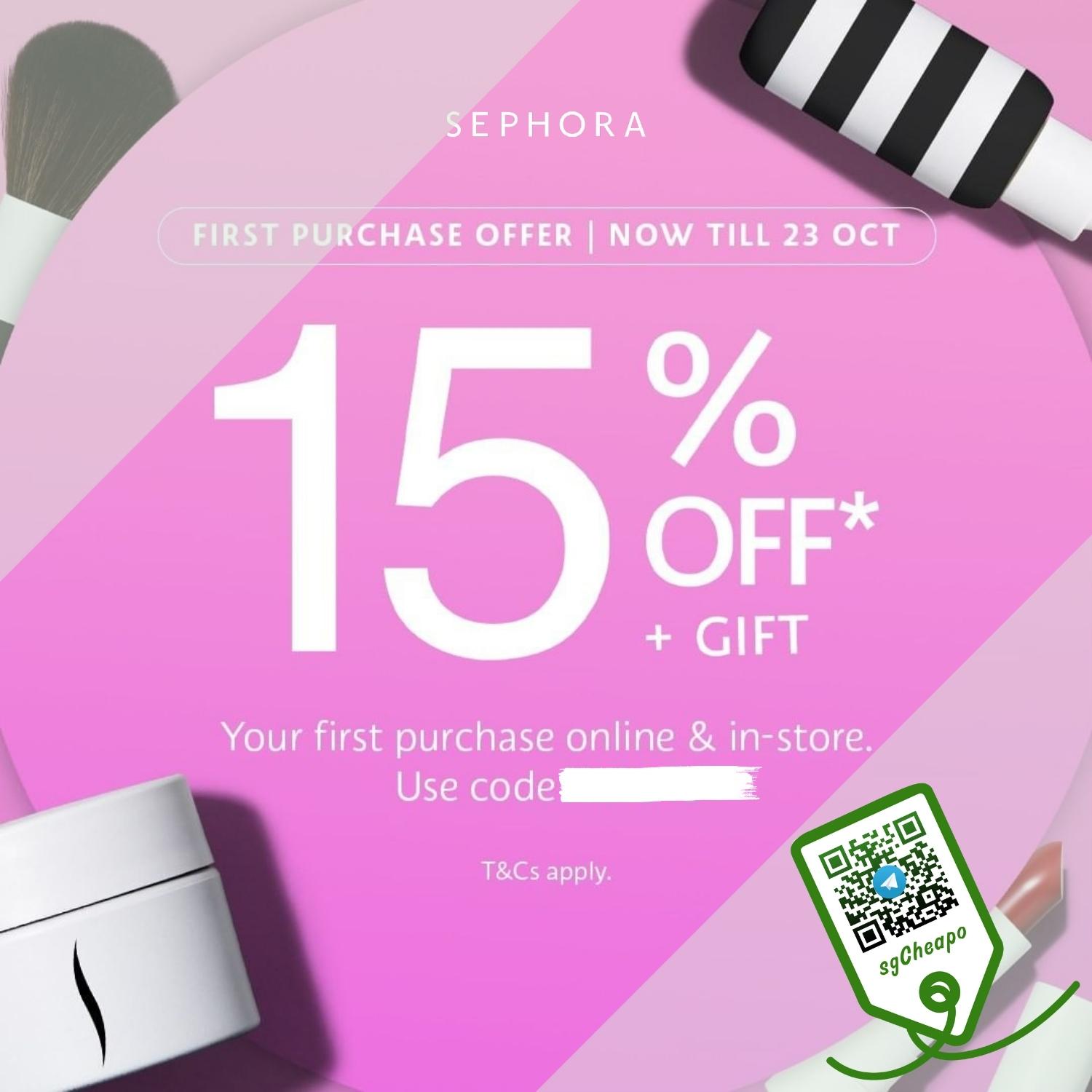Here is a more polished and detailed caption for the advertisement:

---

This image is an advertisement for Sephora, showcasing a special offer for first-time purchasers. The top of the advertisement prominently displays the Sephora brand name, followed by the announcement: "First Purchase Offer - Now Till 23 October," with "Till" spelled as "T-I-L-L." The highlight of the ad is emphasized in very large font: "15% OFF + GIFT," marked with an asterisk next to "OFF."

Below this bold statement, the text reads: "Your first purchase online or in-store," urging customers to use a promotional code (which is unfortunately scratched off in the image) while noting "T&Cs apply."

The background features various makeup items in appealing shades of pink. Notably, there are black-and-white striped makeup applicators and a makeup brush. A white container appears in the bottom left corner, and a lipstick with its top sits in the bottom right corner. A white tag edged in green with an attached QR code and a label detailed "S-G-CHEAPO" dangles from the applicator, secured by a green tie.

--- 

This detailed caption describes the visual and textual elements of the advertisement accurately.